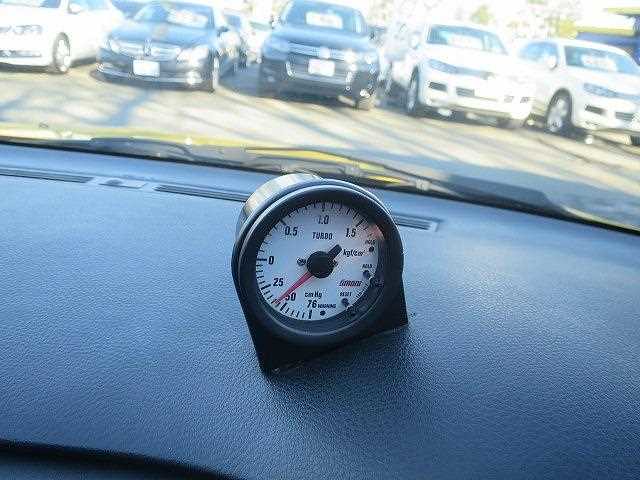The image provides a view from inside a car, looking outward through the front windshield. At the bottom of the frame, the car's dashboard is visible, characterized by its shiny black, grainy texture. Centered on the dashboard is a gauge labeled "Turbo," also marked with "KG." The gauge features numerical increments including 76, 50, 25, 0, 0.5, 1, and 1.5, with five ticks between each main number.

Just above the dashboard, the windshield wipers are noticeable. Beyond the wipers, the road pavement is visible, creating a horizontal line across the image. The background includes several cars: a white car at the top left, followed by a dark-colored car, another dark car in the middle, a white car next to it, and another white car at the far top right corner of the picture.

For further information, visit www.FEMA.gov.